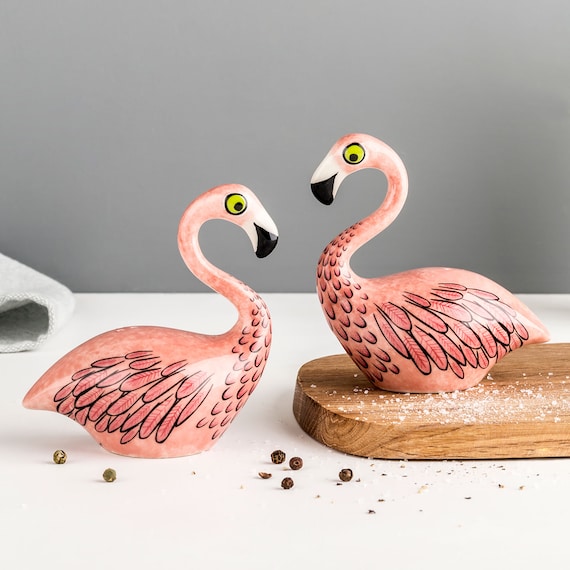The photograph captures a detailed indoor scene featuring two small, vividly painted flamingo figurines, which likely serve as decorative salt and pepper shakers. The square image, measuring approximately four inches by four inches, is neatly divided with a white table or countertop occupying the bottom half and a gray painted wall forming the backdrop in the upper half.

Prominently positioned at the center of the table is a light gray or white fabric napkin. To the left, a striking pink flamingo with a black-tipped beak and a characteristic yellow iris around its black pupil stands out, its body festooned with detailed feather patterns, possibly glitter or glossy paint enhancing its shine. This flamingo sits directly on the white tabletop amidst a scattering of crumbs.

To the right, a second flamingo faces left and is elevated on an oblong wooden cutting board or serving dish. Surrounding this figurine is a sprinkling of what appears to be salt or possibly powdered sugar, with additional whole peppers lying on the table surface beneath, giving the impression of a playful yet elegant table setting. The contrasting placement of the flamingos and the sprinkled materials around suggest a whimsical, artful display rather than any culinary application.